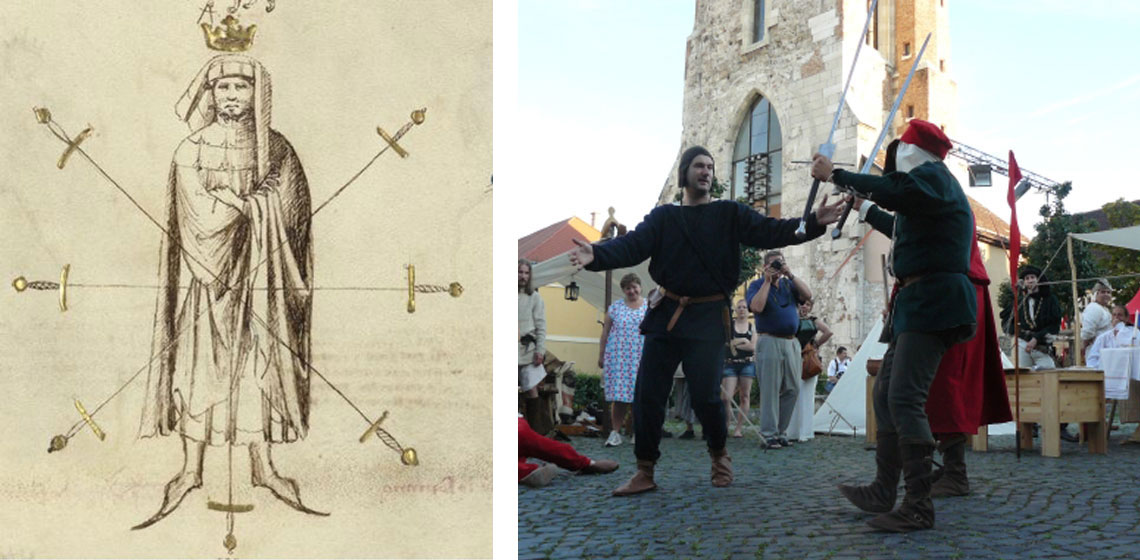In the composite image, the left side features an aged, yellowed drawing of a person adorned in a white turban, a crown, a long robe, and pointy shoes, surrounded by an intricate snowflake-like pattern formed by six crisscrossed swords. This black-and-white illustration has an ancient, worn appearance. On the right side, a photograph displays an outdoor scene with an old, beige cathedral showcasing ornate architecture in the background. In the foreground, two men are locked in what appears to be a staged sword fight. The man on the left wears all black with a hat, a belt, brown shoes, and wields a silver sword. The man on the right, dressed similarly in black, sports a red cap and also brandishes a silver sword. The scene, likely a tourist attraction due to the presence of onlookers, includes another figure in the background capturing the action with a camera.